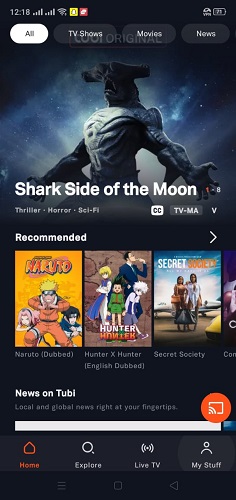This screenshot, taken from a phone at 12:18, displays various icons indicating two wireless signals, a Wi-Fi signal, and a battery at 25%. At the top of the screen, there are four buttons: "All" (highlighted), "TV Shows," "Movies," and "News" (all not highlighted). Below these buttons, there is a promotional image featuring a creature. Overlaid text in large white font reads "Shark Side of the Moon." Next to it, a small "8" is visible. Underneath the title, the genres are listed: "Thriller, Horror, Sci-Fi," along with icons for closed captioning (CC), a TV-MA rating, and a "V" suggesting violence.

Further down, under the "Recommended" section with a right arrow, three items are partially visible. The first title, difficult to read, appears to be "Karuid" or something similar. The second is clearer: "Hunter X Hunter." The third title starts with "Secret," likely "Secret Society." Additional text confirms the availability of "Naruto Dubbed," "Hunter X Hunter English Dubbed," and "Secret Society."